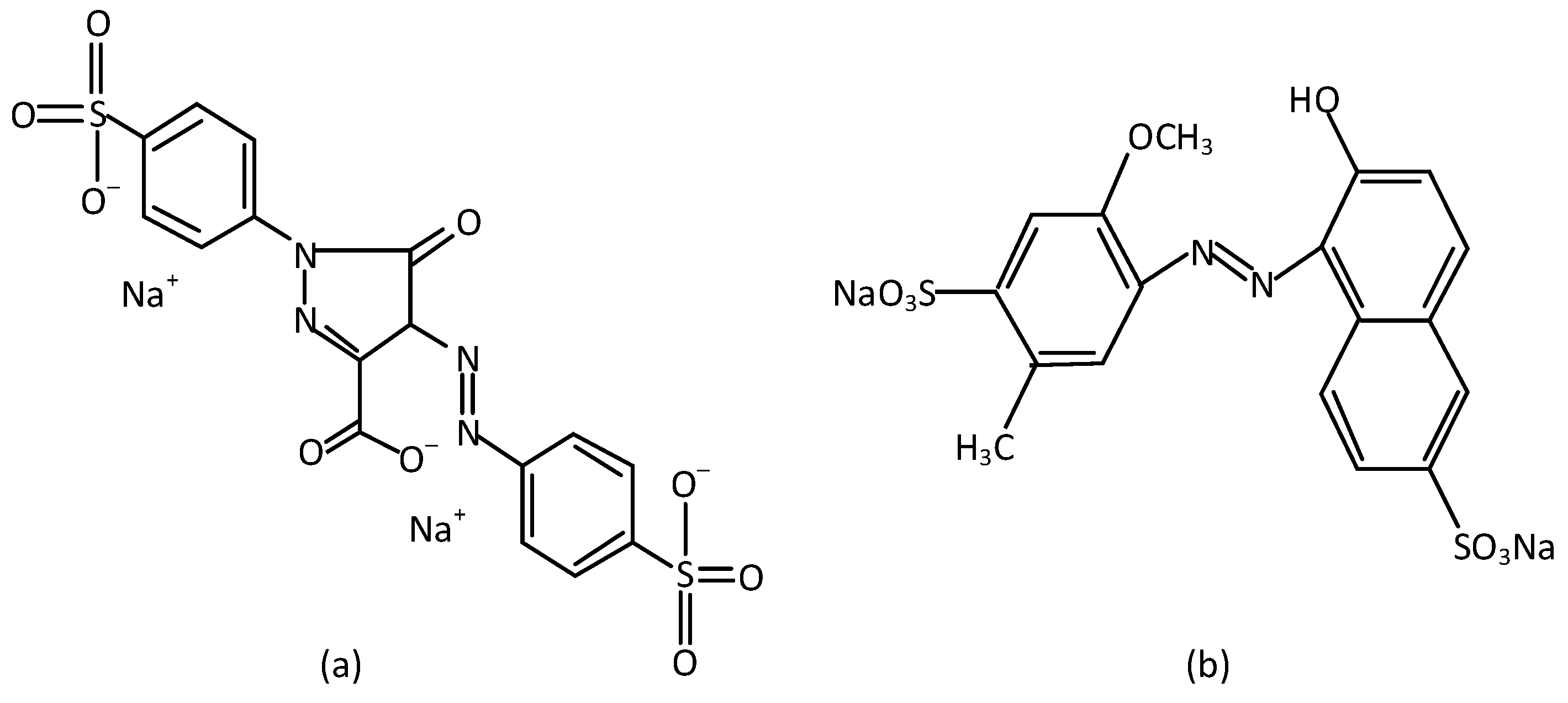In this image, we see two distinct molecular structures labeled as (A) and (B) in black text without the word "figure." The left side (A) features a molecular structure with multiple hexagon shapes, indicating aromatic rings, and various elemental symbols: Na for sodium, O for oxygen, S for sulfur, and N for nitrogen. The right side (B) displays another molecular structure with a formula that includes Na, O₃S, H₃C, OC, H₃, and HO, along with two nitrogen atoms and the compound SO₃Na at the bottom. The image is in black and white, presenting a simple but detailed illustration of these chemical entities, likely useful for chemists to analyze.